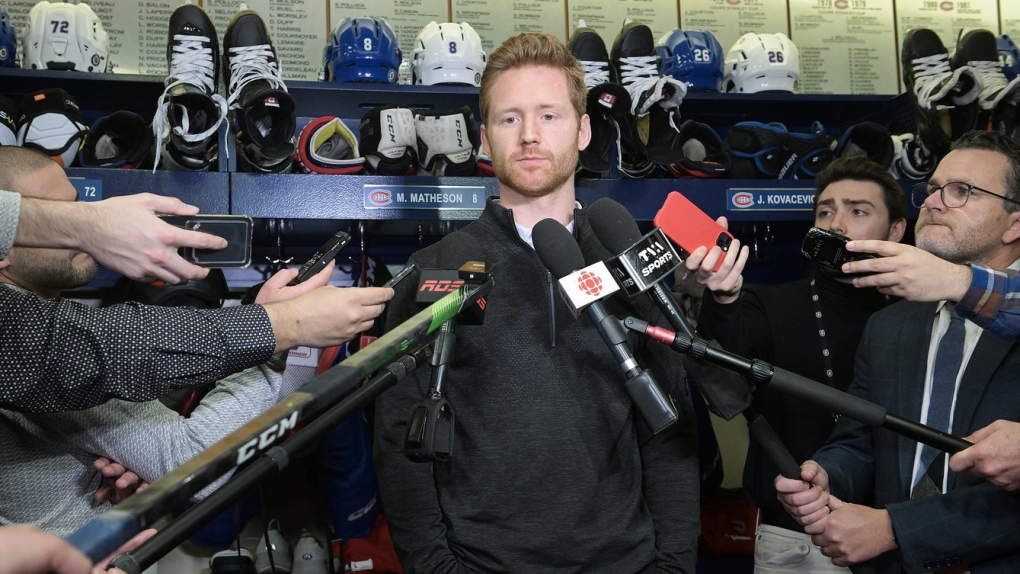The photograph depicts a scene in a men's locker room, likely associated with a sporting event, where a man with short red hair, a stubble beard, and mustache is being interviewed by numerous members of the press. He is dressed in a black long-sleeve coat over a white shirt and is facing forward towards the cameras. Surrounding him are various microphones, small recorders, and smartphones, including one with a red case. Different microphones are visible, with some bearing legible text like "ROS" and "TNA Sports." Behind him, metal shelves hold an array of sports equipment, including small helmets, large shoes, skates, and protective pads, all labeled with name tags and plaques. Despite the absence of a clearly identifiable team name in most descriptions, one mentions Matheson from the Montreal Canadiens, along with the name Kovacek and the number 72 near his locker. Reporters encircle the man, including one with a boom mic and another utilizing a hockey stick outfitted with a microphone, highlighting the intense media coverage.